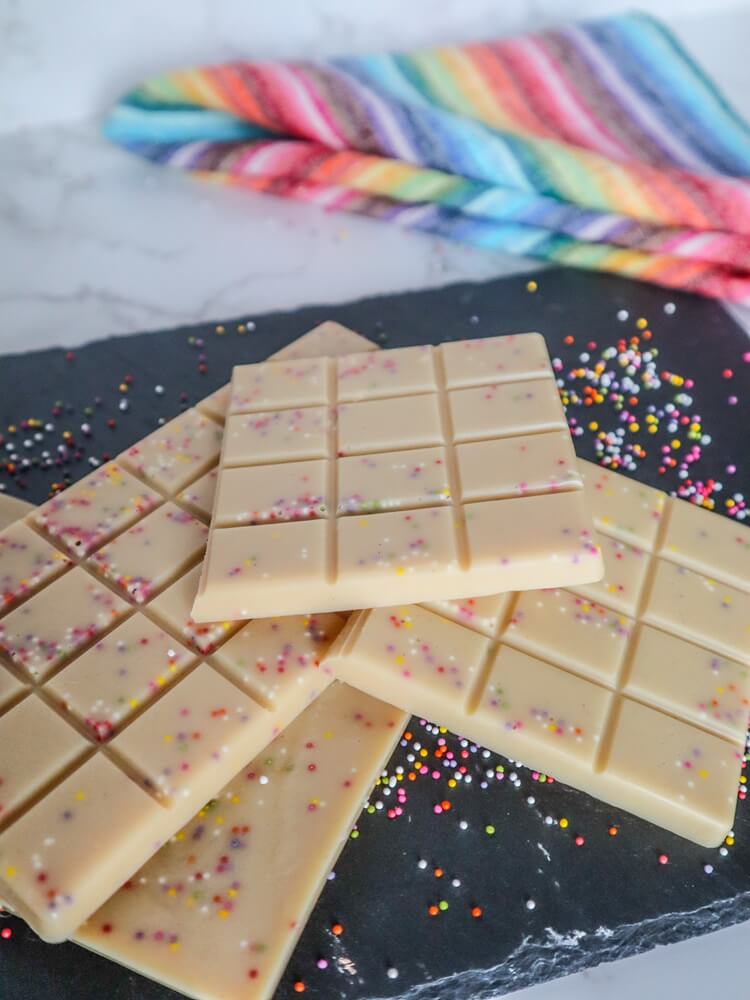The photograph features a close-up view of white chocolate bars adorned with colorful, round sprinkles embedded within the chocolate and scattered around them. These chocolate bars are segmented into small squares, with some pieces showing a grid of 12 squares and others appearing to form larger sections of up to 24 squares, though some are broken, making the count unclear. The bars rest on a black or dark gray slate surface, which, in turn, is placed on a marble countertop. In the background, a vibrant cloth with rainbow stripes—red, green, purple, orange, and blue—is visible, adding a splash of color to the overall composition.